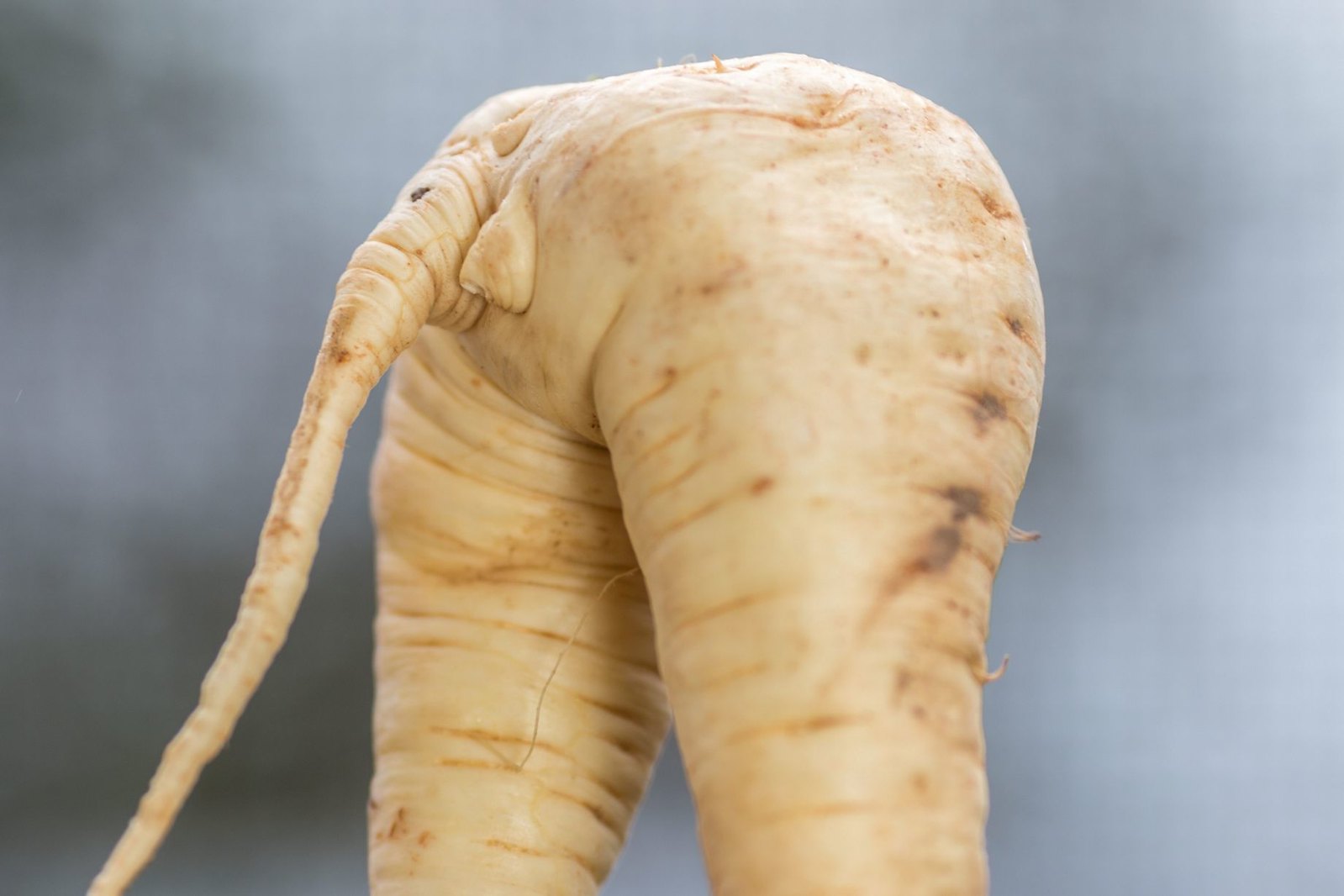The image is a close-up of a peculiar white vegetable that resembles a daikon radish but displays an unusual shape. It appears to be two parts connected together, giving it a deformed look akin to a split carrot or a turnip with dual stalks. The vegetable's form has been compared to human legs or an elephant's trunk, complete with smaller protrusions that might suggest a trunk, a pair of legs, and even rudimentary facial features. The surface of the vegetable is marked by horizontal lines, wrinkles, indentations, and small brown imperfections, including dirt spots from its time in the ground. The background of the image is gray-white and blurry, lending a smoky, indistinct backdrop to the detailed, textured subject of the photograph.